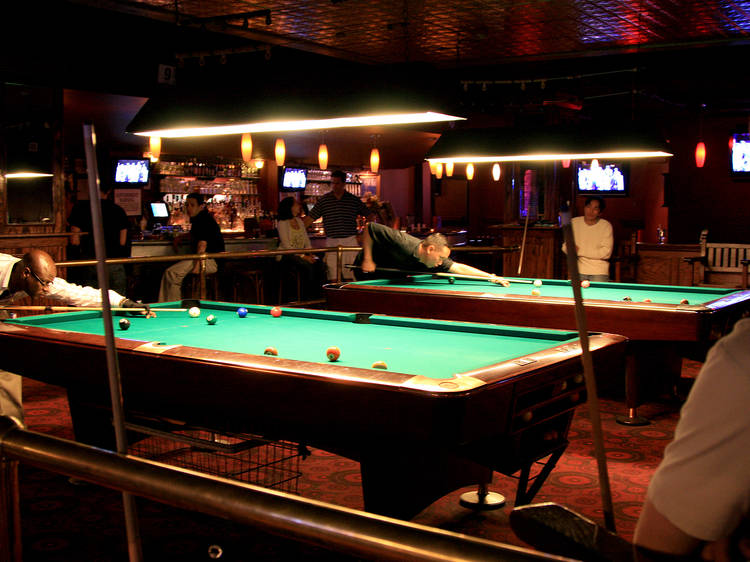In the dimly lit ambiance of a bar, a scene unfolds with two large pool tables covered in green felt, positioned side by side on a red carpeted floor. Rectangular lamps hover over each table, casting focused light on the surfaces where two men are intently lining up their shots. The black male on the left and the white male on the right are each poised over their respective pool cues, deep in concentration. Surrounding them, the pool area is elegantly enclosed by a golden gate, separating it from the rest of the bar.

In the background, the bar itself is a hub of quiet activity, with a few patrons seated and engaging in conversation, their faces illuminated by the warm glow of small, oval-shaped orange lights that line the room's textured, reflective ceiling. One man in a white shirt stands alone, watching the games unfold, while another stands closer to the pool area, partially captured in the foreground, holding or resting beside a pool cue. On the left-hand side, another cue leans against a railing, ready for its next use.

Adding to the lively yet cozy atmosphere, several television monitors are mounted, likely broadcasting a sports game, while a variety of glasses and bottles are neatly arranged behind the bar. This scene, a blend of leisure and focus, is a snapshot of an evening in a bar where the camaraderie of pool and the shared enjoyment of sports come together.